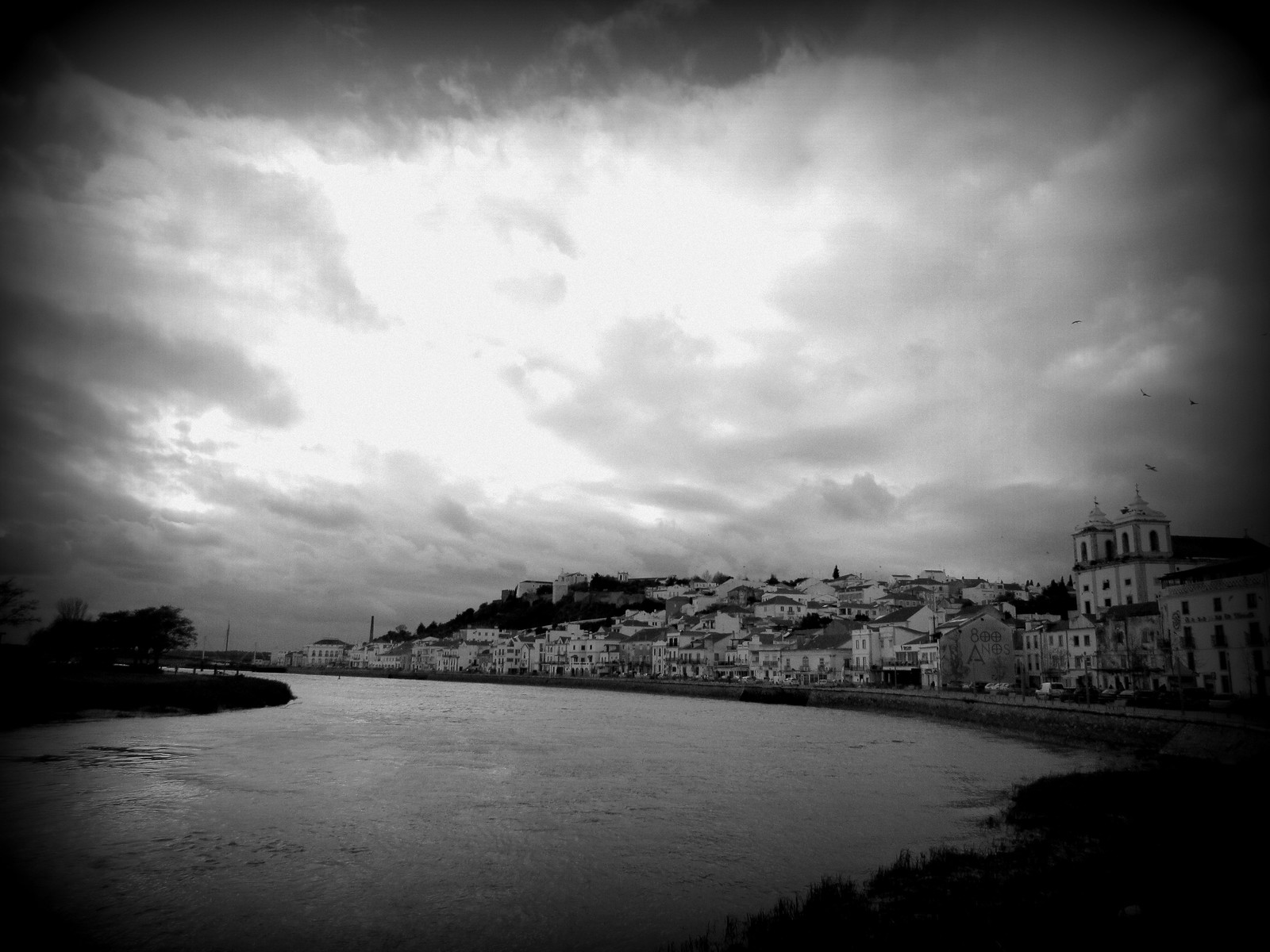This black and white photograph captures an overcast outdoor scene of a European city, likely in Spain, judging by the "800 años" sign visible on one of the buildings. The city, characterized by Moorish architecture, stretches along a large river. On the left side of the image, several white buildings are stacked on a hill, reflecting the region's historical architecture. In the foreground, grassy patches can be observed, leading to a body of water that runs parallel to the cityscape. The right side of the picture features birds flying in the distance, adding a dynamic element to the serene landscape. The sky, heavily clouded with only faint sunlight peeking through, dominates the upper half of the picture, creating a somber yet captivating atmosphere.